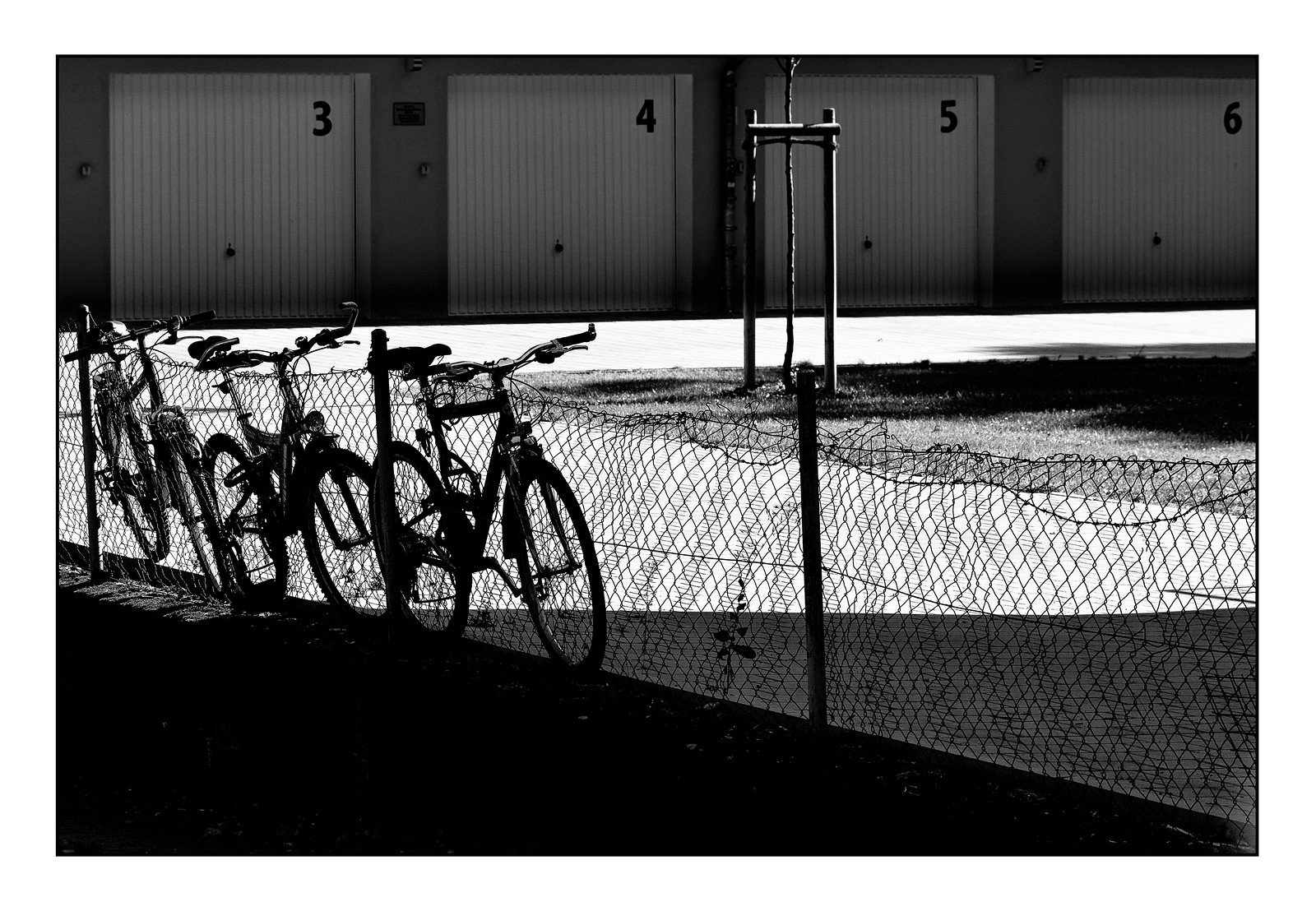This black and white photograph captures a scene with four large, numbered garage doors labeled three, four, five, and six, arranged from left to right. The doors are painted white and are part of a dark gray building, giving a stark contrast in the monochrome setting. The pavement in front appears bright, indicating sunlight hitting the scene, particularly on the left-hand side, while shadows cast near the grass in front of doors five and six add depth to the photo.

In front of these doors, there is an old, weathered chain-link fence running vertically across the image. Three black 10-speed mountain bikes, with their tires firmly on the ground, lean against this fence. The image's mid-section showcases a small patch of short, dark grass, suggesting its green hue in a color photo. A thin tree grows from this grassy area, extending vertically upwards, adding an element of nature to the industrial backdrop.